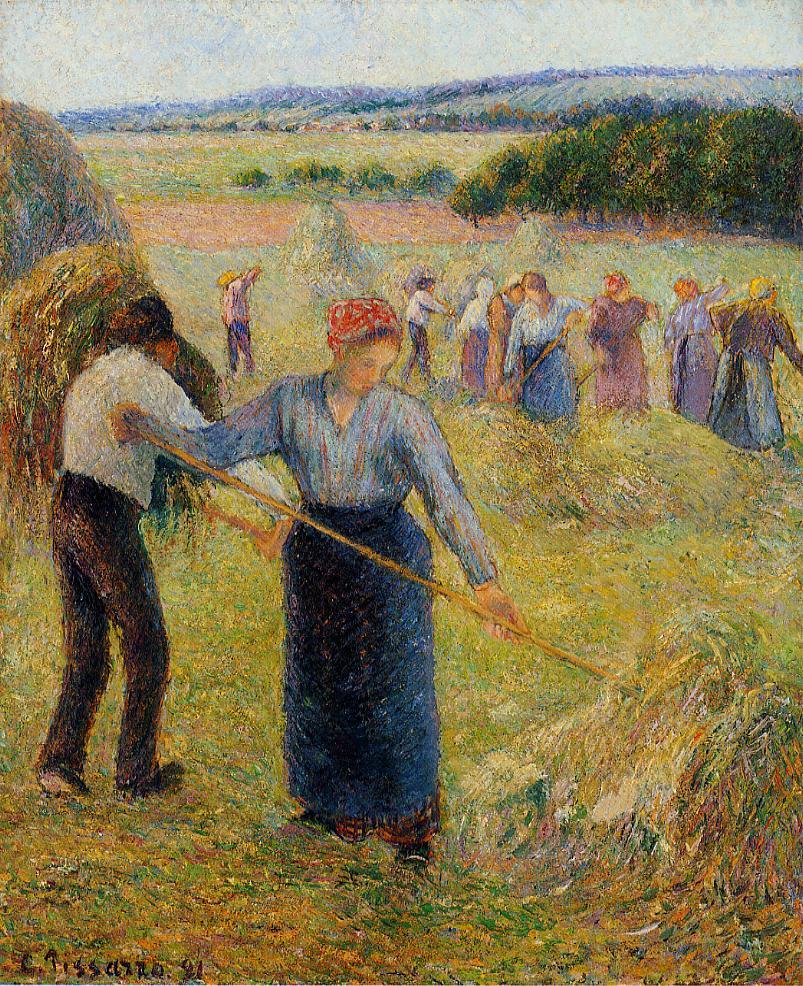This painting, signed in the bottom left corner "C. Toscaso, 91," vividly depicts a bustling threshing scene set in a vast field. Dominating the foreground is a woman engaged in raking hay. She is detailed with a long blue skirt and a matching long-sleeved top featuring orange stripes, and she wears a red handkerchief on her head that partially conceals her short brown hair. She stands poised with a rake in her hand, next to a low-lying pile of hay.

Adjacent to her, with his back turned, is a man dressed in black trousers and a white long-sleeved shirt, similarly holding a threshing pole. These two figures are surrounded by a multitude of women, all involved in the laborious task of gathering hay. The women are adorned in various hues of blue and purple dresses, many also wearing handkerchiefs, some of which are red.

The expansive landscape is painted with predominantly green and brown tones, featuring a scenic backdrop of trees, grass, and mountains. In the distance, there is a grove of dark green trees on the right, with a more sparse arrangement of greenery towards the center, indicating a well-worked field. Beyond these elements, the painting captures additional layers of horizon, concluding with a modestly ascending mountain range under a soft blue and white sky. The scene conveys the active, communal effort of threshing in a serene, rural setting.